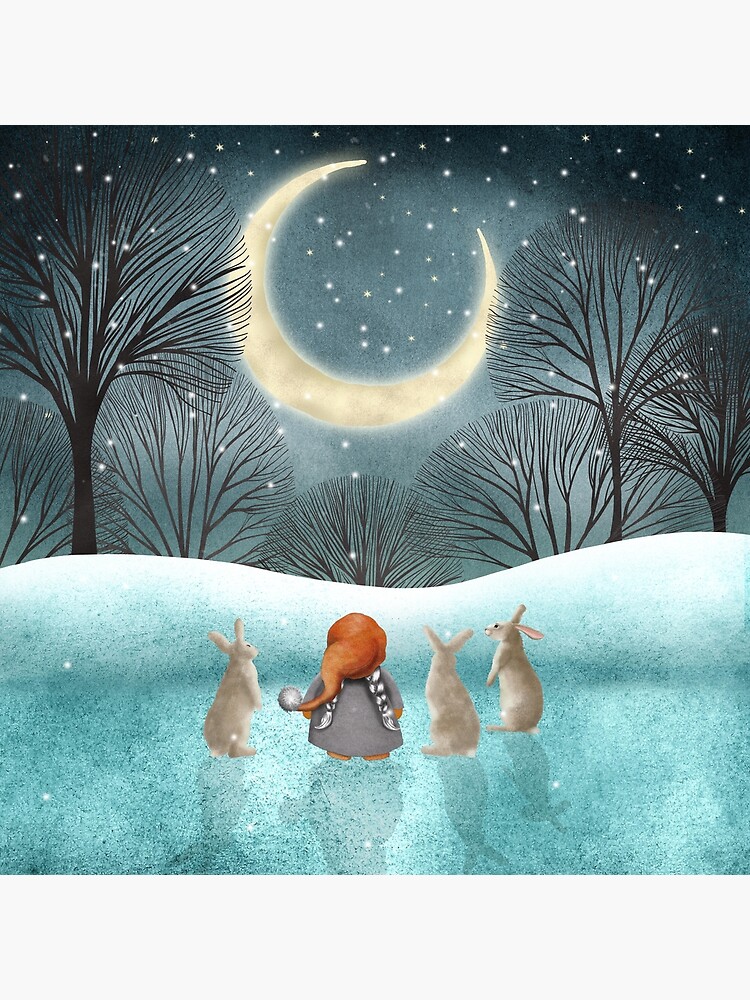The illustration, likely from a children's book, vividly portrays a serene night scene with a rich, dark blue sky dotted with bright white stars and a prominent crescent moon glowing with a yellow hue at the top center. The foreground features a snow-covered hill, tinted with blue, where a little girl, or perhaps a gnome, stands alongside three upright rabbits. The girl wears an orange hat with a white fuzzy ball on the tip, a hooded jacket, and a scarf. They all gaze upwards at the night sky. The scene is framed by seven bare winter trees with dark brown, fan-like branches that surround the moon, adding a sense of wonder. Shadows of the figures stretch behind them on the snow, which glistens brightly even in the cold, snowy night. The tranquil beauty and detail of the scene evoke a sense of quiet curiosity and enchantment.